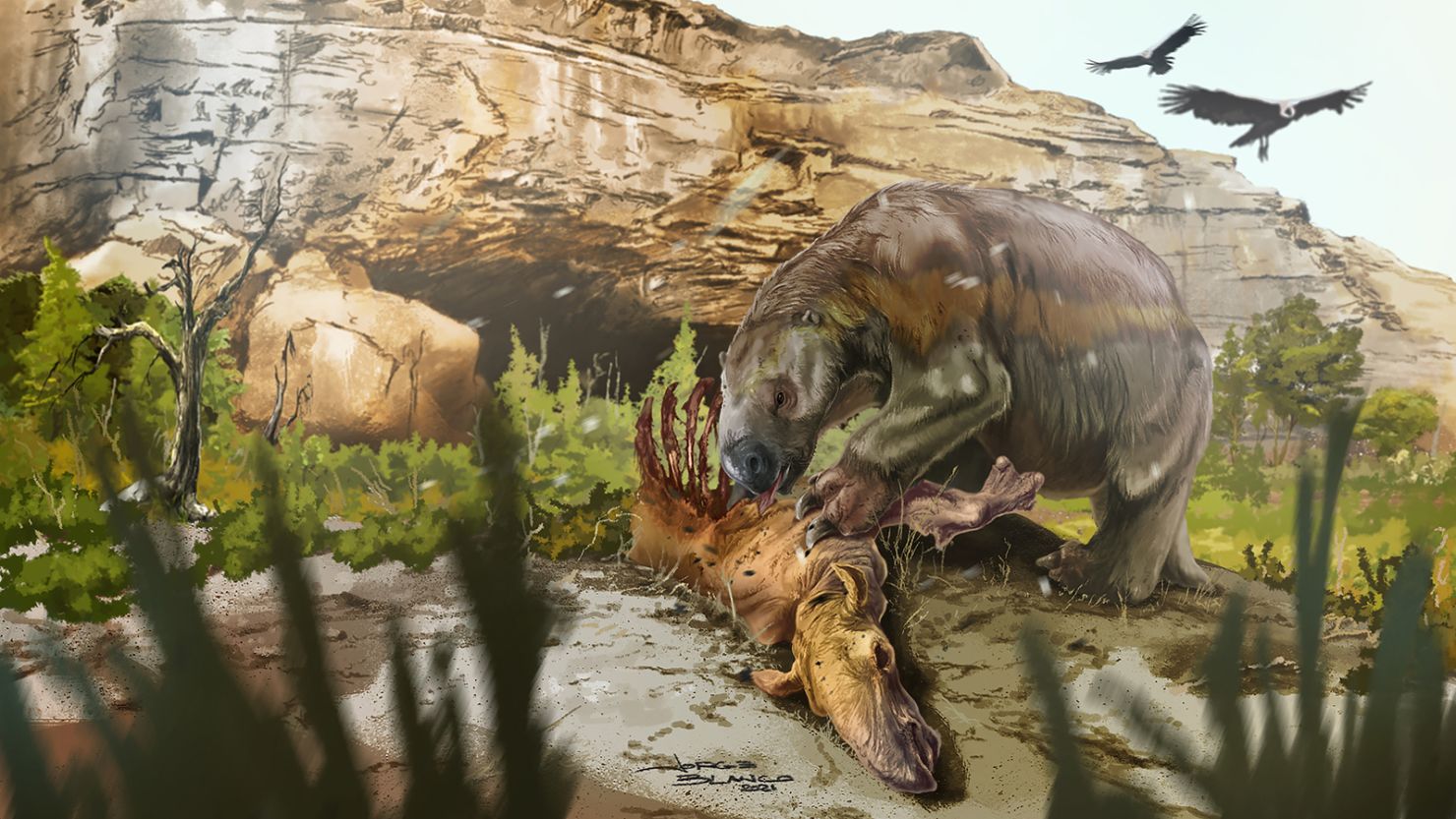In this detailed painting, an artist’s conception depicts a prehistoric mammal, blending characteristics of a sloth and a grizzly bear, tearing apart and feasting on a proto-moose carcass. The creature, with a bear-like face and broader, clawed toes, features a brown top coat transitioning to lighter and greenish-brown hues. Its pointed nose and large paws add to its distinctive look. The scene is enriched by two large, poultry-like birds - one resembling a condor with wattles and another in the distance that could be mistaken for a bald eagle - circling overhead. The background is dominated by rugged, tall, rocky cliffs and a leafless tree, while the foreground is framed with bushes, grasses, and other blurred foliage. The artist’s signature, though small and indistinct, adds authenticity to the evocative piece, making it a vivid window into a prehistoric world.